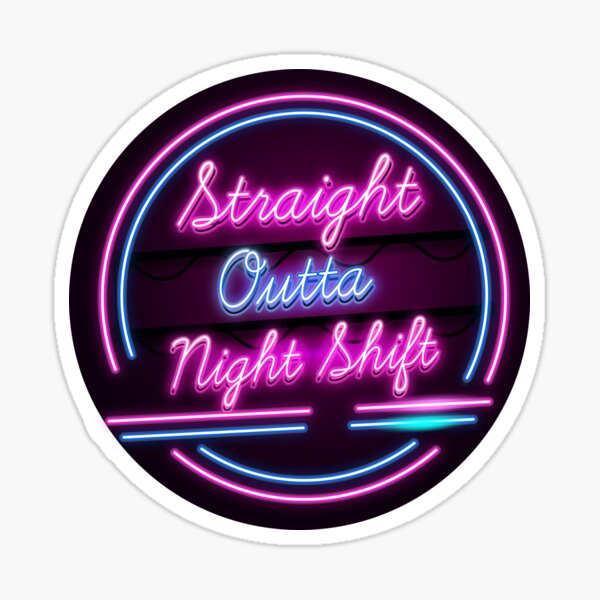The image depicts a vibrant neon sign resembling a large diner clock. The sign features a white outer border encircling a dark interior. Within this circle, several neon elements are arranged in a structured and aesthetic manner. A cursive purple neon line arcs slightly over half the circle horizontally, followed by a blue neon line underneath and another quarter-circle neon blue line. These lines are layered with a final purple circle segment completing the neon arc design. Center-aligned on this neon backdrop, large, glowing cursive text displays the words "straight" in purple, "out of" in blue, and "night shift" back in purple, spread over three separate lines. This creates a cohesive and striking visual against the sign's dark circle interior, making the text pop as if viewed through neon-lit slats or blinds. The entire composition rests over a light blue background, adding an extra layer of visual contrast.